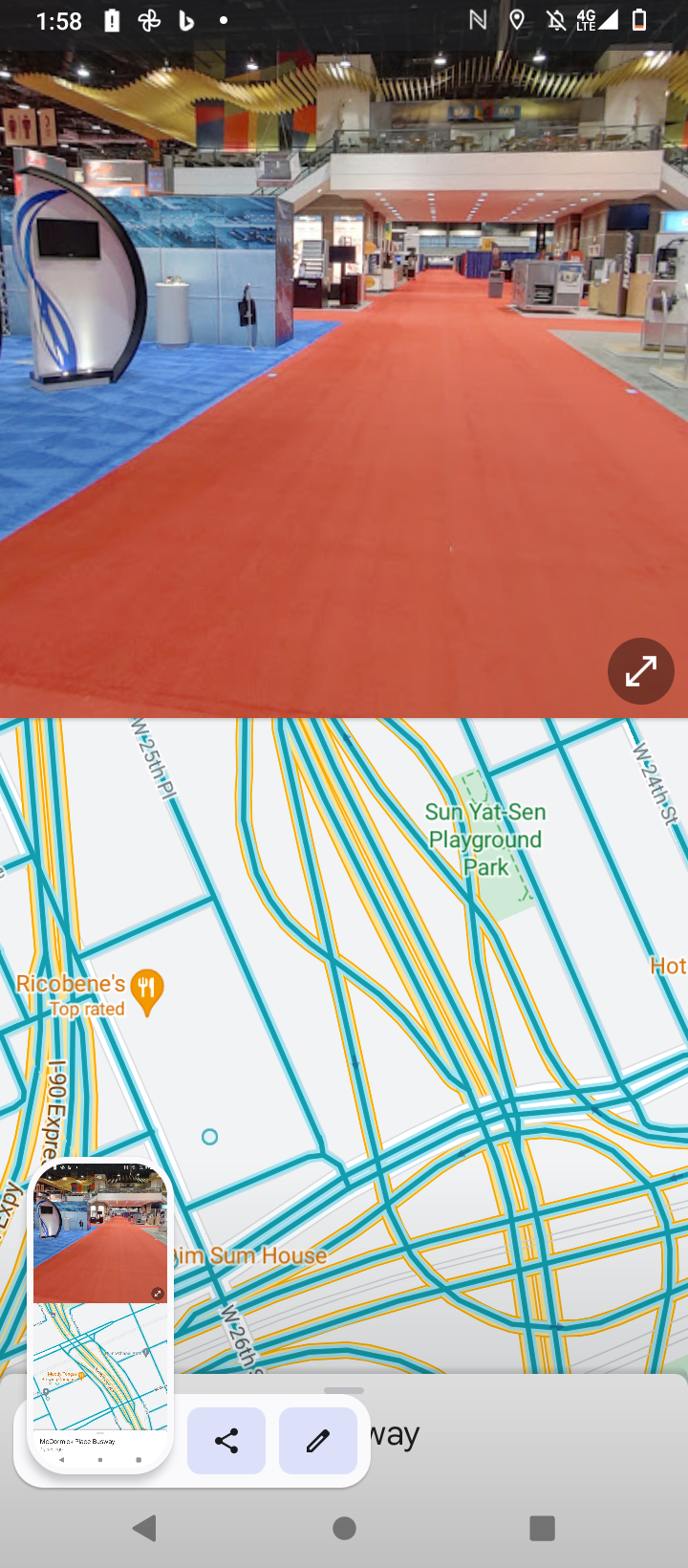The image is divided into two sections, one above the other. The top section is a screenshot from a phone showcasing an extravagant event, possibly an industry expo. The scene is set under a sprawling canopy, with a vibrant red carpet that extends far into the distance. On the right-hand side, there is a prominent stand featuring a large white structure with a screen and blue stripes. Scattered throughout the venue are various exhibition stands inviting attendees to explore, potentially collect promotional items, and enjoy complimentary beer.

The bottom section of the image displays a detailed map, likely from a navigation app such as Google Maps. The location seems intricate, with a complex network of roads and pathways. A notable point on the map is a playground area named Samyeolsan, suggesting the setting could be either China or Korea. The map currently doesn’t display any active route, focusing instead on providing comprehensive geographical information.